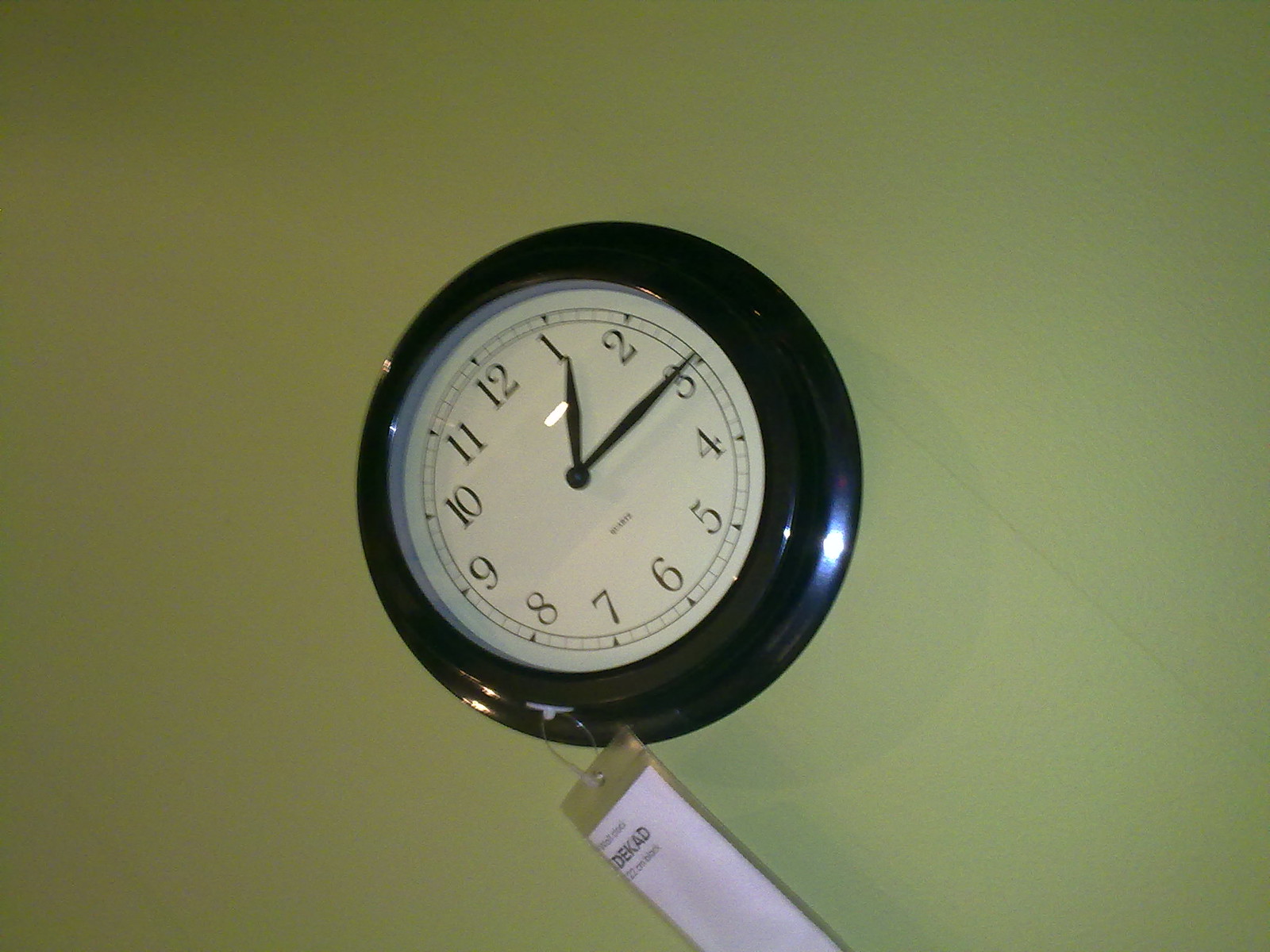This photograph features a circular, older-style clock mounted on a wall, which is a shade of olive or moss green. The clock has a black metal housing and a white face, protected by a glass cover. The black numbers and hands—absent of a second hand—indicate the time, which is approximately 1:15, though the minute hand is slightly off from the 3, suggesting it could be closer to 1:14. Surrounding the face are inner rings with minute markings. Attached to the left side of the clock is a gold and white plastic tag, possibly a store tag from IKEA, with "DEKAD" written in black text, hanging by a plastic zip tie. The clock's overall aesthetic combines the vintage charm of its design with practical modern elements like the informative tag.